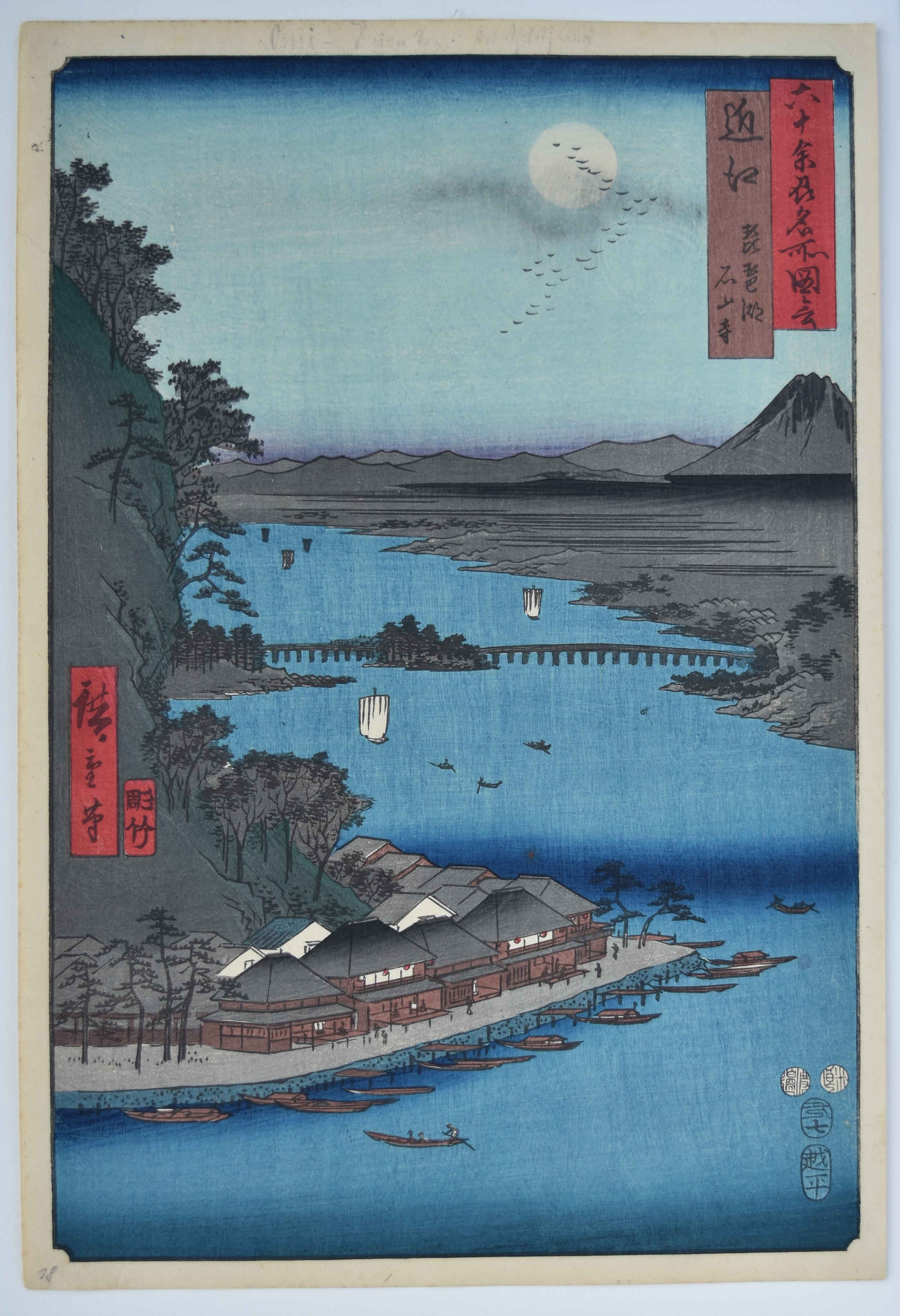This intricate Japanese-style artwork, displayed on a pristine white surface, captivates with its detailed depiction of a tranquil riverside village. Nestled along the shore towards the center-left, the village is framed by a towering mountain that cradles the quaint wooden buildings, which align harmoniously with the coast. The foreground is animated by a cluster of small wooden fishing boats, while tiny figures dot the landscape, adding a sense of scale and life.

In the midground, several sailboats traverse a serene river, contributing to the scene's peaceful ambiance. A gracefully arched bridge spans the water, connecting the left mountain shoreline to a central island, and onward to the right shoreline, creating a sense of interconnectedness within the landscape.

Dominating the background, a majestic volcanic peak rises steeply from the earth on the right, contrasting with a series of smaller mountains arrayed to its left. The sky above is adorned with a luminous moon, beneath which a flock of birds form a perfect V, enhancing the composition's sense of movement and tranquility. This artwork masterfully blends natural and man-made elements, evoking a serene and harmonious atmosphere.